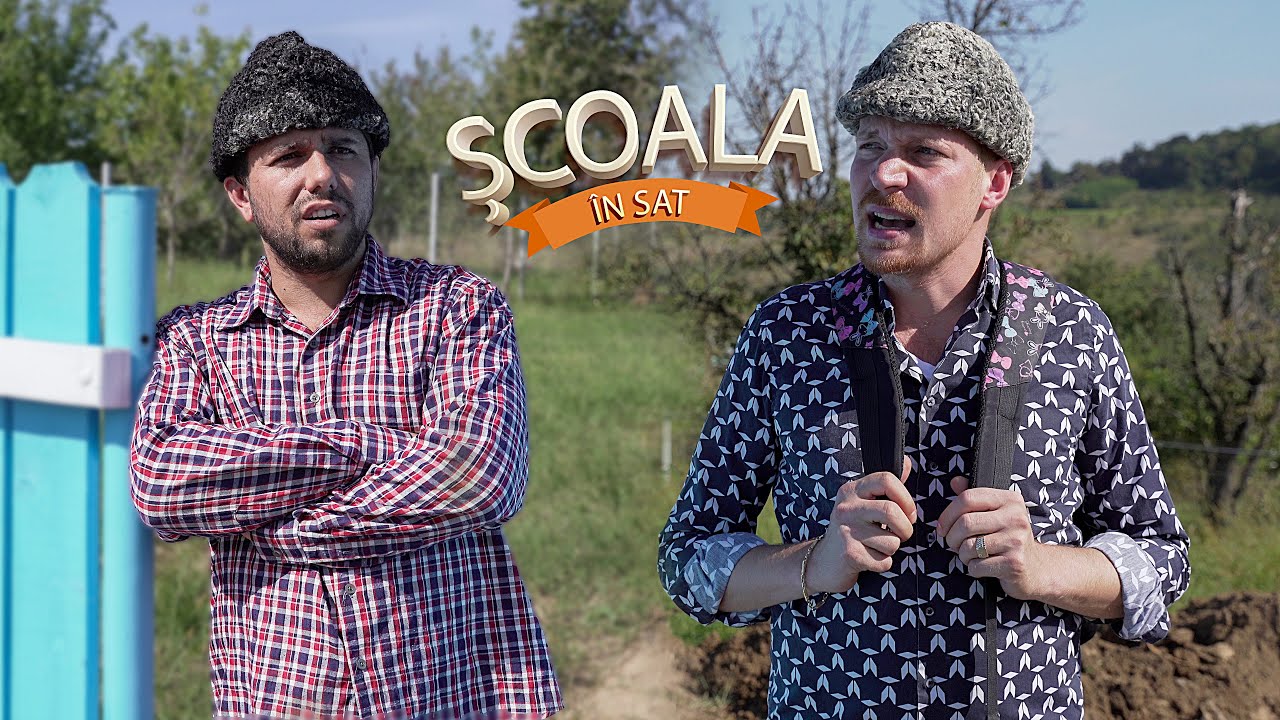In this image, two men stand outdoors, possibly in a yard, with a light blue fence on the bottom left. Both men are centered in the picture and are wearing wool hats—they both also have button-down shirts, though the colors and patterns differ: the man on the left wears a flannel shirt with a purple, red, and white checkered pattern, while the man on the right dons a navy shirt decorated with white objects, possibly flowers. The man on the left leans against the fence and has his arms crossed, while the man on the right, who appears to be talking, holds onto his backpack straps, which feature flower designs. Above and between the men, an orange banner bears the text "Skwala Nsat" in white. The background includes green trees, foliage signaling a spring or summer day, and a clear blue sky. The overall scene captures a moment of interaction, possibly in a foreign land, given the unusual text and the eclectic apparel. The image is vibrant with colors such as blue, gray, white, orange, red, purple, black, and light blue, enhancing the outdoor setting.